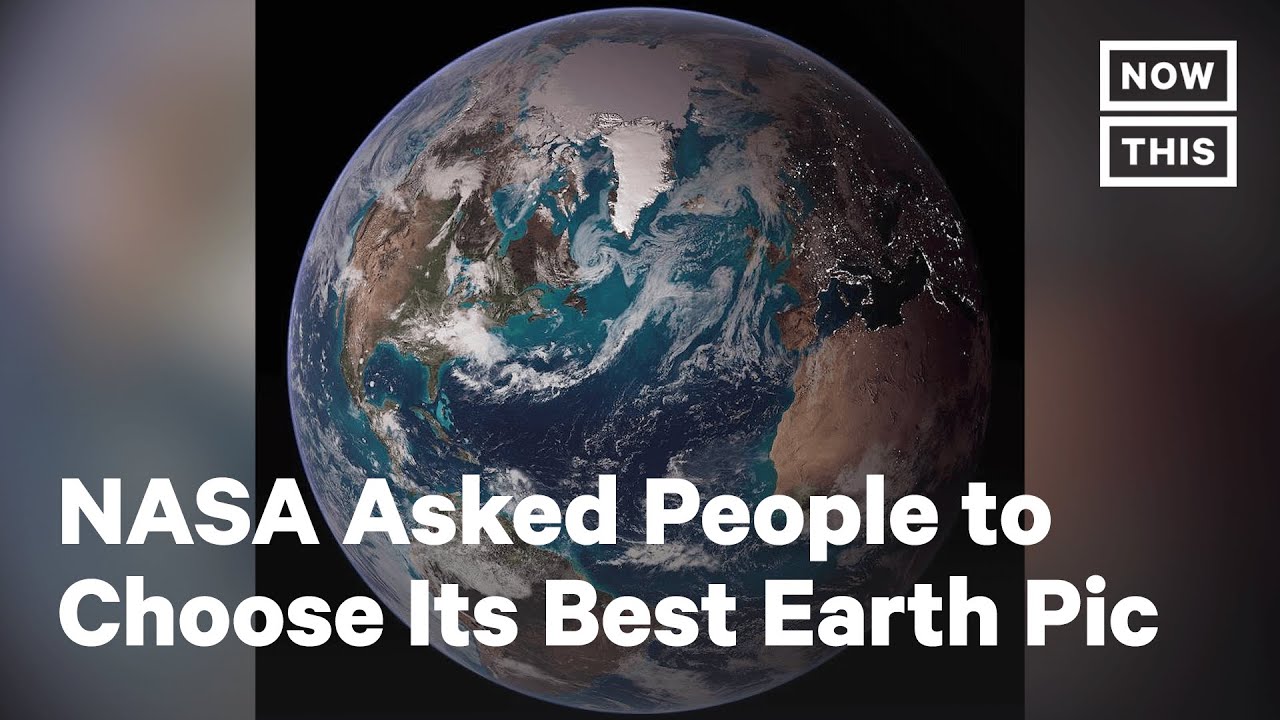The image is depicted within a rectangular layout divided into three segments. The central segment prominently features a breathtaking view of Earth from space, with swirling clouds and vibrant landmasses visible. Flanking this central segment are two narrower bands, each displaying a blend of muted colors: shades of stormy blue, soft pink, and patches of white, creating a serene and atmospheric backdrop.

In the top-right corner of the image, there's a smaller box with a thick white border. Inside, the word "NOW" is displayed in bold, white capital letters against a darker background. Directly below this, an identical box contains the word "THIS" in the same style, resulting in a combined message that reads "NOW THIS."

The main focal point of the rectangle is the text spanning the width of the central segment, which reads: "NASA ASKS PEOPLE TO CHOOSE ITS BEST EARTH PIC." Key words in this statement are emphasized with capitalized letters: "N-A-S-A", "ASK", "PEOPLE", "CHOOSE", "BEST", "EARTH", and "PIC," ensuring the viewer's attention is immediately drawn to these important aspects of the message.